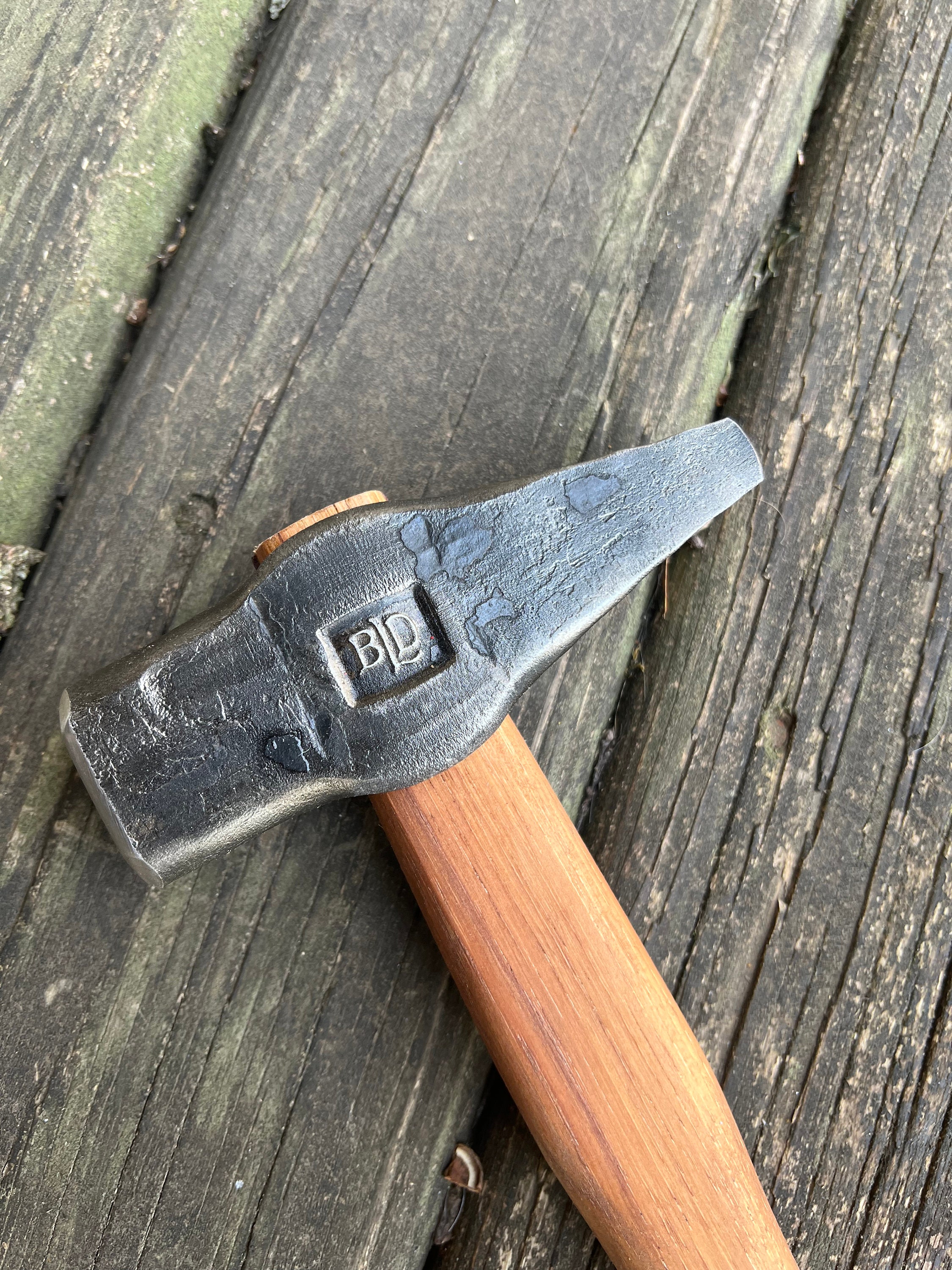The photograph is a close-up of a hammer meticulously resting on a weathered wooden surface, likely an outdoor patio or picnic table based on the visible moss accents. The photograph itself is rectangular, with the length twice that of the height. The hammer takes center stage, focused on its head while the wooden handle extends diagonally from the bottom right up towards the middle.

The hammer head is made of wrought iron, featuring a silverish-black hue marred by numerous dents and spots that suggest a handmade quality rather than a machine-made finish. It showcases a distinctive design: a square-shaped front facing the left and a triangular-shaped backside pointing to the top right. The handle, exhibiting a polished wooden texture, intriguingly peeks out from the top of the head, which is an unusual feature.

A raised leather mark is present where the handle connects to the head, inscribed with the letters "BLD"—presumably the manufacturer's logo. The wooden planks beneath the hammer are dark gray with prominent mossy spots, adding an earthy, aged ambiance to the scene. The sunlight reflects off parts of the hammer, indicating the photograph was taken on a sunny day, further emphasizing the rustic outdoor setting.